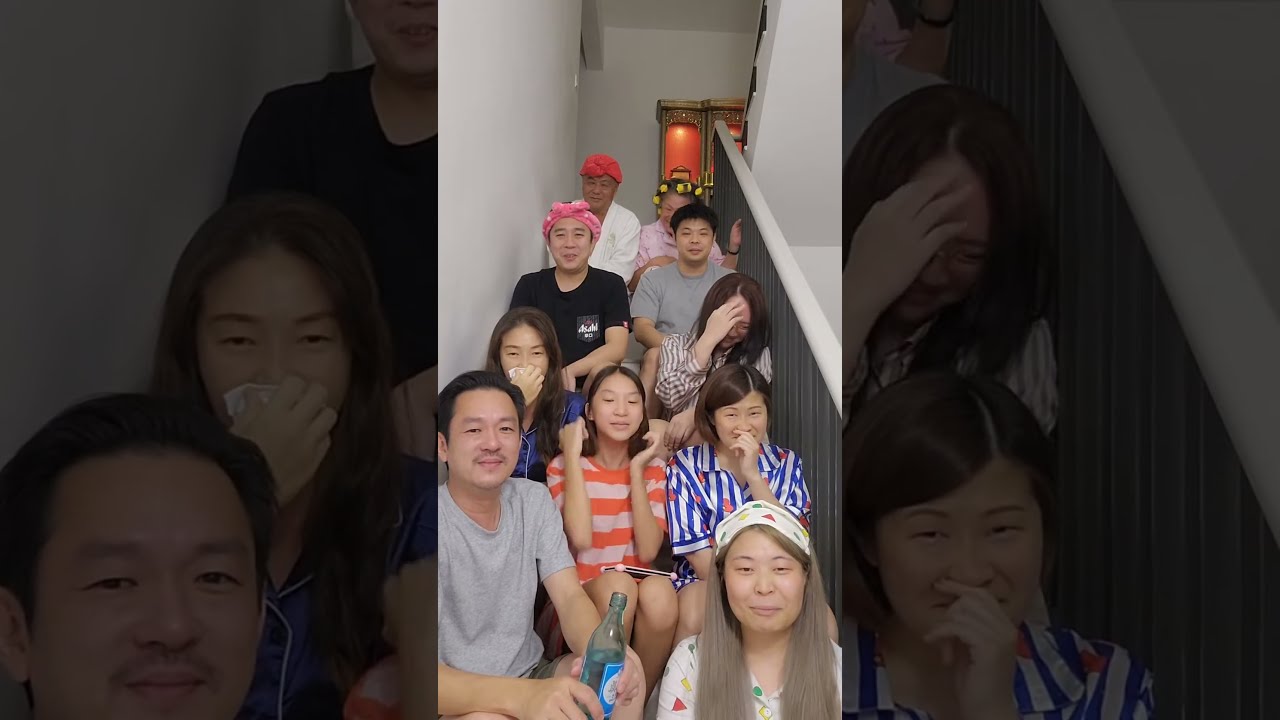This photograph captures a lively and intimate moment of ten Asian individuals, predominantly older, posing on a stairwell. The image is taken from a low angle, looking up the steps, creating an inclusive portrait of friends or family members enjoying their time together. The group radiates joy and amusement, with many of them smiling broadly. 

At the forefront, a man with his eyes closed and a smirk on his face holds a bottle of water, surrounded by several women. He is flanked by a lady with very long hair and a scarf on her head. Behind her, another woman, dressed in a striped pajama top, is laughing and partially covering her mouth with her hand. Beside her, another woman in an orange and white striped top sits cheerfully. Further in the background, a person with rollers in her hair adds to the jovial atmosphere. The stairwell's white walls contrast with the gray and white stair banister, while a small shelf at the back painted orange with gold trim adds a splash of color. The photograph's composition is narrowly framed with borders on the left and right made up of enlarged and grayed-out sections of the central image, emphasizing and framing the cheerful group sitting on the steps.